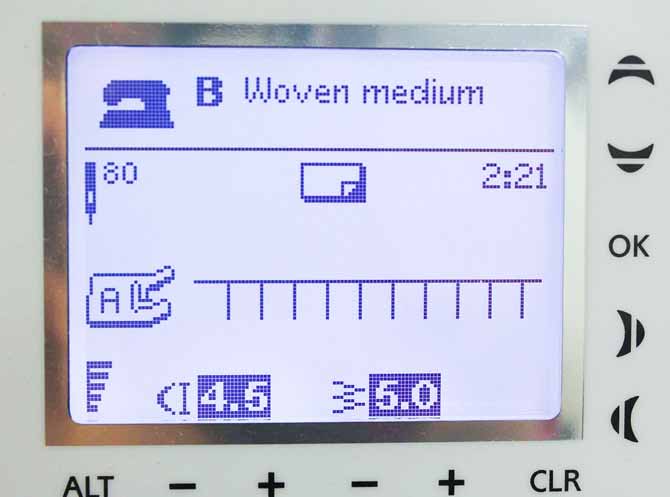The horizontal rectangular image showcases an LCD display for a sewing machine, surrounded by a gray, functional touch-control panel with directional buttons for up, down, left, and right, as well as commands for OK, ALT, plus, minus, and clear. The central screen, rimmed by a silver border, features a bluish display where various pieces of data are shown. At the top, it prominently displays the words "woven medium" next to a small pixelated image of a sewing machine. Nearby, a large letter "B" indicates a mode or selection, and beside it is a needle icon labeled with the number "80". To the right, the time is displayed as "2:21". Additionally, the screen shows details of the selected stitching pattern—depicted as a straight stitch with specific tension settings marked at 4.5 and 5.0. Overall, the display offers an intuitive user interface with clear visual indicators and numerical data pertinent to sewing machine adjustments.